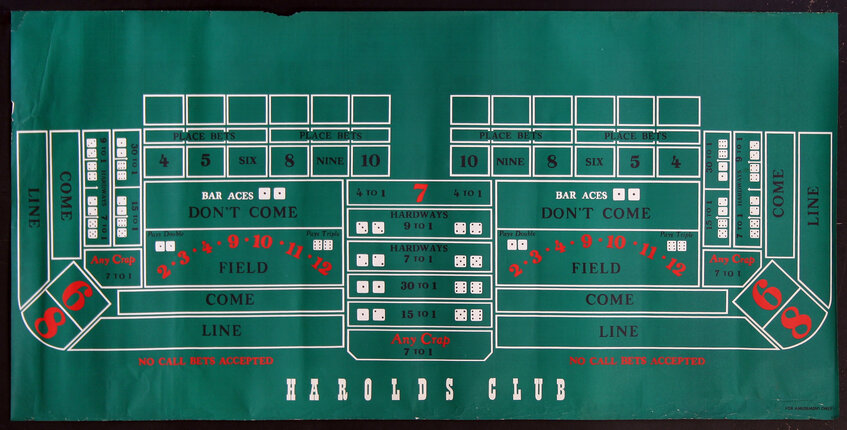This image depicts a detailed betting diagram for a dice game, likely craps, with a green background labeled "Harold's Club." The diagram features numerous text annotations and numbered squares, indicating various betting areas and game instructions. Key sections include "Place Bets" at the top, "Come Line," "Don't Come," "Field," "Bar Aces," "Any Crap," and a note at the bottom reading "No Call Bet Accepted." Prominent numbers such as 4, 5, 6, 8, 9, and 10 are displayed, with large red numbers 6 and 8 in the bottom corners and a central number 7. The image appears as if it's a wrinkled piece of green cloth, typical of a craps table layout, laid flat and featuring multiple dice illustrations showcasing various dice rolls.